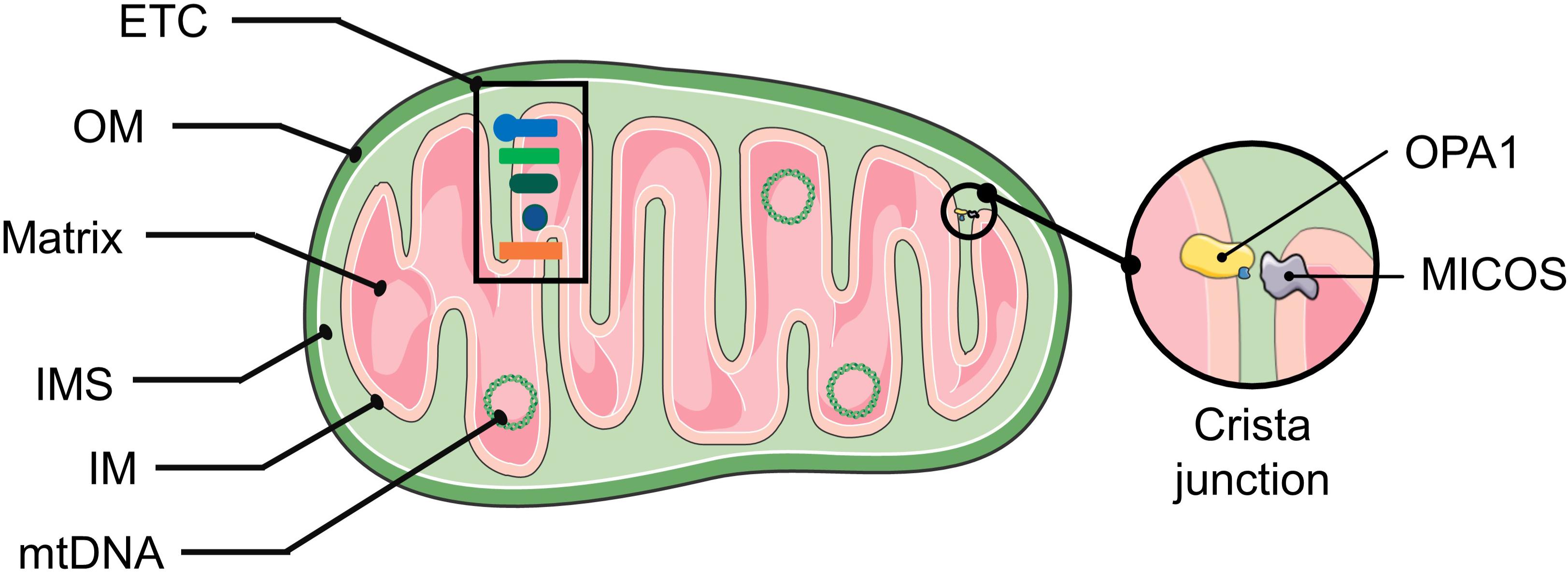This detailed illustration appears to be designed for an educational science poster, possibly for use in a biology classroom. The main focus is a green oval shape positioned on the left, representing a cellular structure, possibly an amoeba. Inside this oval is a complex, pink, zigzagging pattern resembling internal organelles or perhaps the cell's digestive system. On the right side of the image, there is a close-up inset labeled "Krista Junction," showcasing a detailed interaction between cellular components. In this close-up, a small yellow structure is shown in close proximity to a gray structure, indicating an area of significant biological activity. Additionally, the diagram prominently features the term "OPA1 in micos," suggesting a focus on specific mitochondrial proteins or gene regulation involved in cellular processes. Annotations on the far left side of the image, with terms such as ETC, OM, Matrix, IMS, IM, and MTDNA, are accompanied by arrows that guide the viewer's attention to corresponding parts of the diagram, likely illustrating various elements and functionalities within the cellular or mitochondrial context.